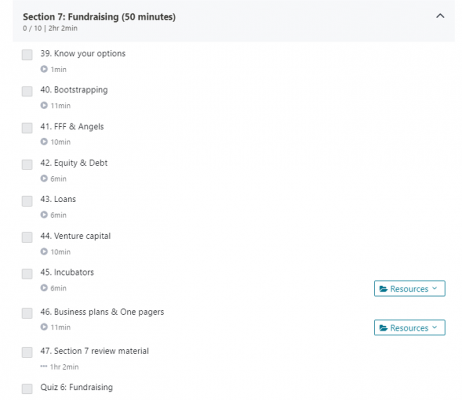This is a screenshot from a computer screen featuring a structured list of video modules related to fundraising, displayed on a clean white background with black and gray text. At the top of the screen, a light gray, horizontal, rectangular bar spans the width, with "Section 7, Fundraising, 50 minutes" boldly written inside. To the far right of this bar, an upward-pointing arrow is present.

Beneath this header, a column of interactive elements is aligned on the left side. Each item in this column begins with a small square checkbox followed by descriptive text, indicating the topic and duration of video modules:

1. "39. Know Your Options, 1 minute"
2. "40. Bootstrapping, 11 minutes"
3. "41. FFF and Angels, 10 minutes"
4. "42. Equity and Debt, 6 minutes"

Next to each topic description is a circular button with a triangle (play icon), signifying that these are videos that can be played by clicking the button.

At the bottom right corner, there are two small, light green boxes labeled "Resources," which are also likely clickable for additional materials or information.